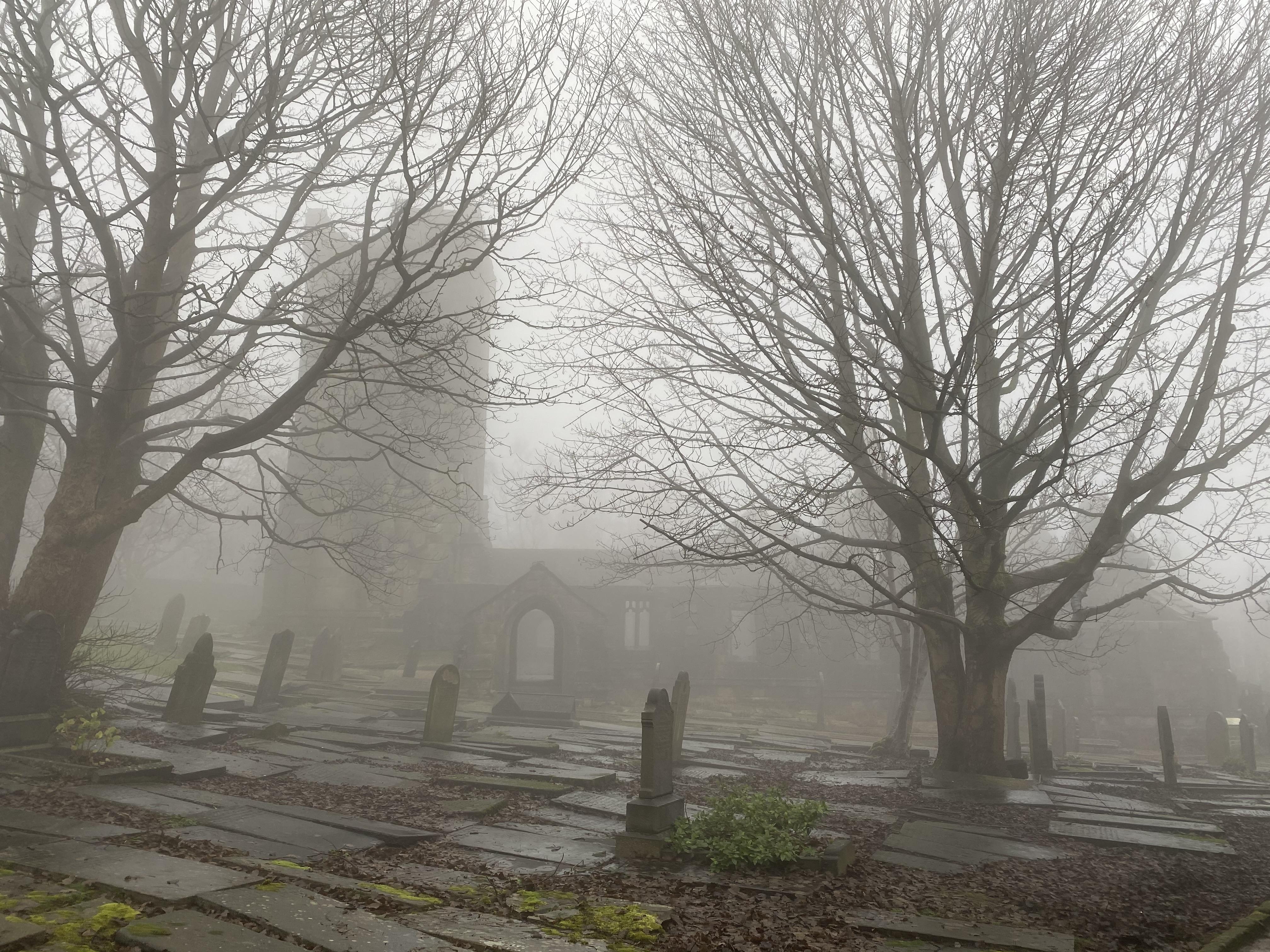The photograph features a moody, atmospheric scene of a cemetery on a very foggy day. Dominating the foreground are numerous headstones and large horizontal concrete slabs covered with fallen, crunchy brown leaves, with only patches of grass visible. The left and right sides of the image are framed by large, bare-branched trees that extend out of the frame, adding to the eerie ambiance. In the background, barely discernible through the dense fog, stands an old, castle-like church. The structure includes an arched entryway and a tall tower on the left, with a lower, rectangular section on the right. The overcast, gray sky and pervasive fog accentuate the haunting, melancholic mood of the scene.